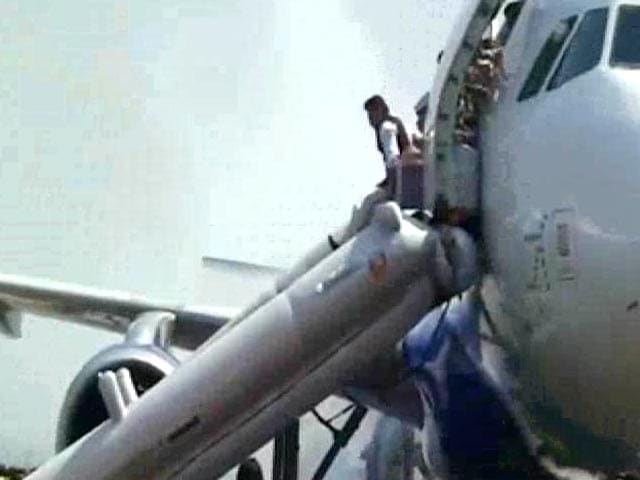The image captures a slightly blurry, close-up side view of an airplane with an open door, from which a passenger is descending down a slide designed for emergency evacuation. The plane's body features a combination of silver and blue, though details are somewhat obscured due to the blurriness. The visible passenger, possibly female, has long brown hair and is dressed in a long-sleeve white shirt paired with a black vest, and is preparing to slide down while a second person holding something stands behind them. Prominent in the upper right corner are two small cockpit windows, and the airplane's wing can be seen in the lower left portion of the frame. The sky dominates the upper part of the image, presenting a cloudy, blue backdrop. The entire scene appears pixelated, making finer facial features and exact details difficult to discern.